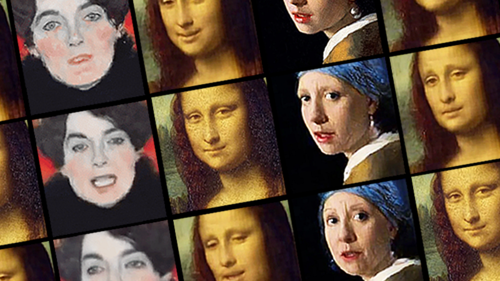This intriguing image showcases a detailed collage that combines digital artistry with classic paintings. Set up in the format of a photo booth strip, the collage consists of four different columns and three rows, displaying a grid of twelve altered artworks. Featured prominently are multiple interpretations of renowned pieces such as the Mona Lisa and Girl with a Pearl Earring. Each column represents a different painting subjected to computerized facial manipulations, presenting varying expressions and emotions.

In the first column, a woman reminiscent of classical portraiture is depicted with three distinct facial expressions, transitioning from a neutral gaze to a candid, slightly open-mouthed look. The second column focuses on the Mona Lisa, presenting her iconic, serene smile, her classic expression, and another version whereby she appears skeptically amused. 

The third column displays three variations of Girl with a Pearl Earring. The original painting is present, followed by manipulated versions where she appears aged and worried, further adding to the dynamic emotional range. The fourth column includes yet another portrayal of the Mona Lisa, with one image missing, and the visible ones showing her with a concerned expression and the original calm demeanor. 

This unique compilation mirrors the fun spontaneity of photo booth snapshots, yet captures the timelessness and depth of classical paintings, making it a captivating and thought-provoking piece.